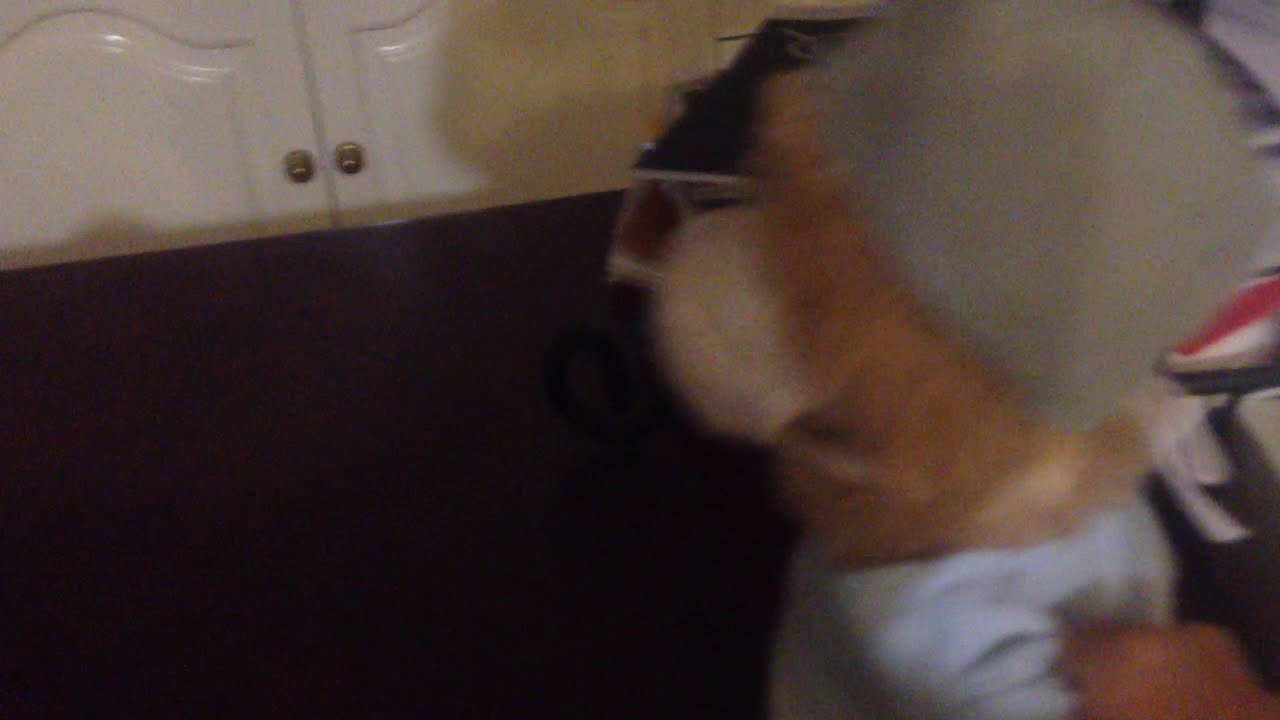In this very blurry photograph, the main focus is difficult to discern due to the poor quality and indistinct elements. However, the most consistent details include a background featuring a white cabinet with two gold handles situated in the upper left portion of the image. Below the cabinet is a dark, predominantly black area that spans the left section of the photo. The centerpiece, while unclear, appears to involve a brown table or surface on the right side, holding various items.

A notable aspect of the image is a stuffed animal adorned in a shirt and a gray hat. A person's hand is partially visible, seemingly grasping the stuffed animal, with a slight emphasis on the shirt. Directly behind the stuffed animal is a stack of notebooks, though this part is not the main focus. Despite the overall blurred quality, these elements stand out and provide some context to the otherwise indistinguishable scene.